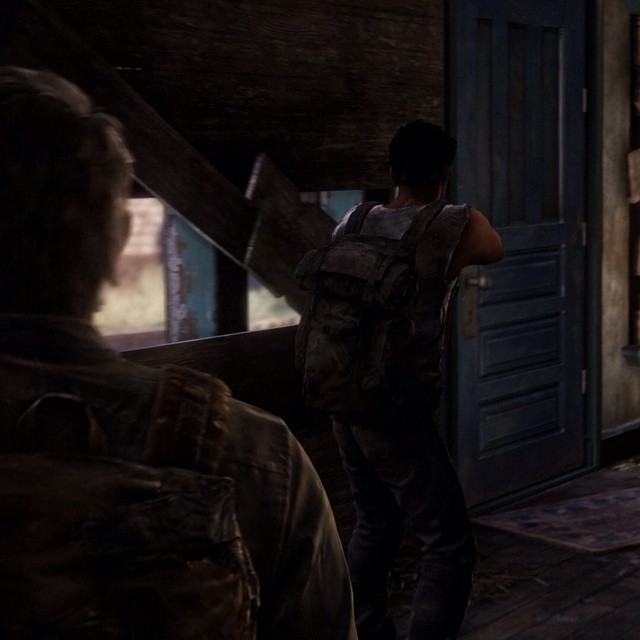In a dimly lit, decrepit room that appears to be abandoned and partially boarded up, two men stand amid the shadows. The atmosphere is reminiscent of a post-apocalyptic video game, with grungy details adding to the eerie scene. The room's focal point is a large, grime-smeared window partially obscured by a haphazard arrangement of wooden boards, leaving a significant gap through which daylight tries to penetrate. The man on the left has his back to us; he sports short brown hair and is clad in a gray denim jacket with a weather-beaten brown leather backpack slung over his shoulder.

Facing him, another man of tan skin and short black hair holds a weapon menacingly in his hand. He wears a dirty gray sleeveless shirt and dark blue jeans caked in grime. Slung across his back is a black, worn-out hiking backpack. To their right, slightly ajar, is a large blue door with a silver knob, barely hanging on its frame. Below this door, an old purple and blue rug lies crumpled and dusty. The right side of the frame reveals a bit of a stained, cream-colored wall, hinting at the room's past. Through the window, the outside world contrasts sharply with the dim interior, as bright sunlight illuminates a blue pillar, patches of green grass, and a distant building.